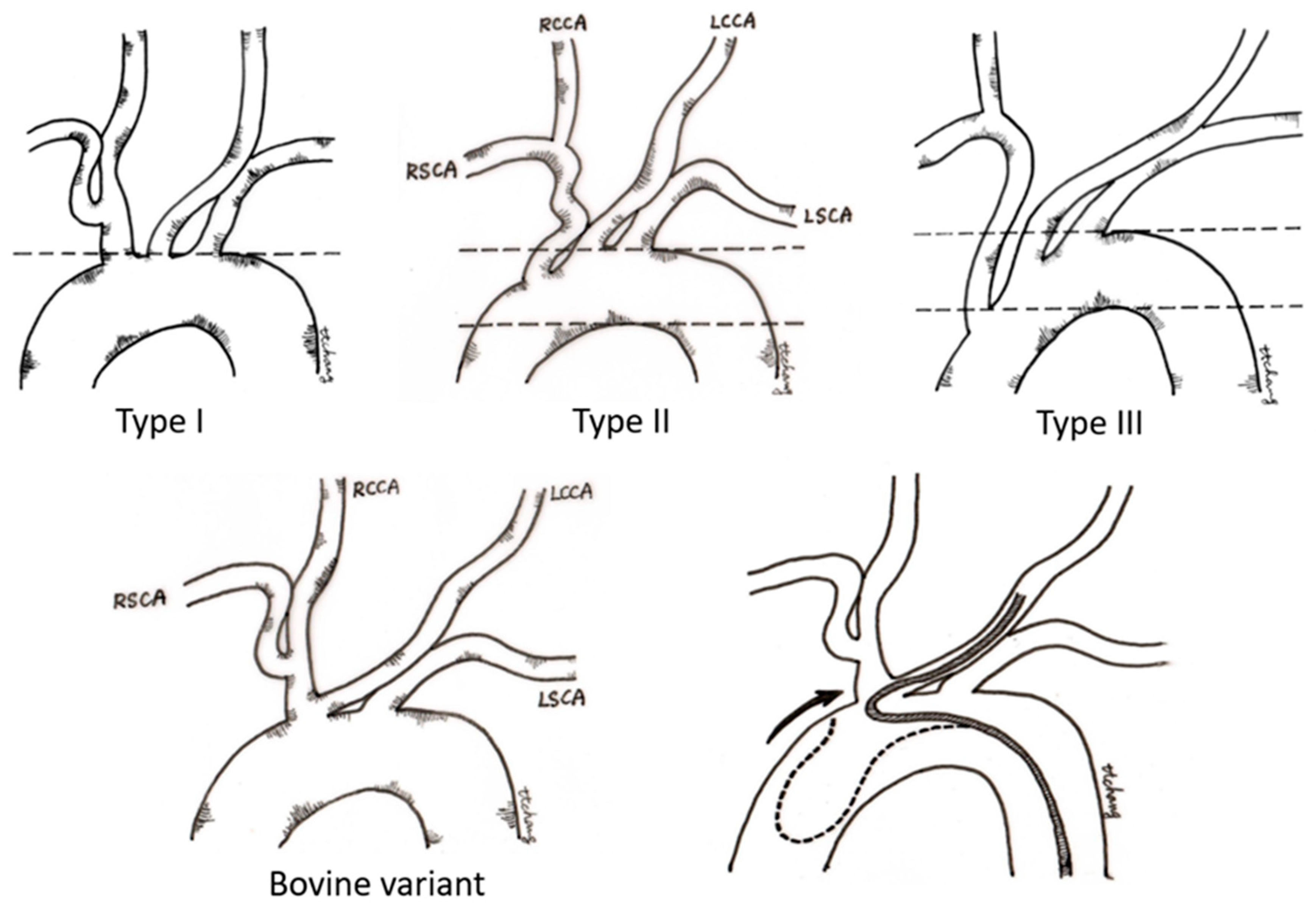The image depicts a series of five black-and-white anatomical diagrams comparing different types of circulatory structures, with varying arrangements and labels. Each illustration features a semicircular base with several tendril-like extensions emerging from it. 

- **Type 1:** This diagram shows an unlabeled semicircular base with four tendrils extending outward.
- **Type 2:** Similar to Type 1, this has a semicircular base but includes labels on each of the four extensions: RSCA, RCCA, LCCA, and LSCA. There are additional dotted lines across and halfway down the semicircle.
- **Type 3:** This retains the dotted lines from Type 2 but features a slight alteration where the leftmost extension protrudes further into the semicircular base. The tendrils remain unlabeled.
- **Bovine Variant:** This diagram omits the dotted lines but follows the general layout of Type 2, with the extensions labeled RSCA, RCCA, LCCA, and LSCA. Significant detail includes the leftmost tendril originating from another tendril rather than directly from the base.
- **Unlabeled (Fifth Diagram):** Similar to Type 3, it shows the same structure, but there is a distinctive black line running from the bottom right of the semicircular base to the second extension from the right, making it appear different from the previous diagrams.

Overall, this detailed comparison highlights variations in the branching and labeling of the circulatory structures, with particular focus on the leftmost extension and the unique black fiber in the final illustration.